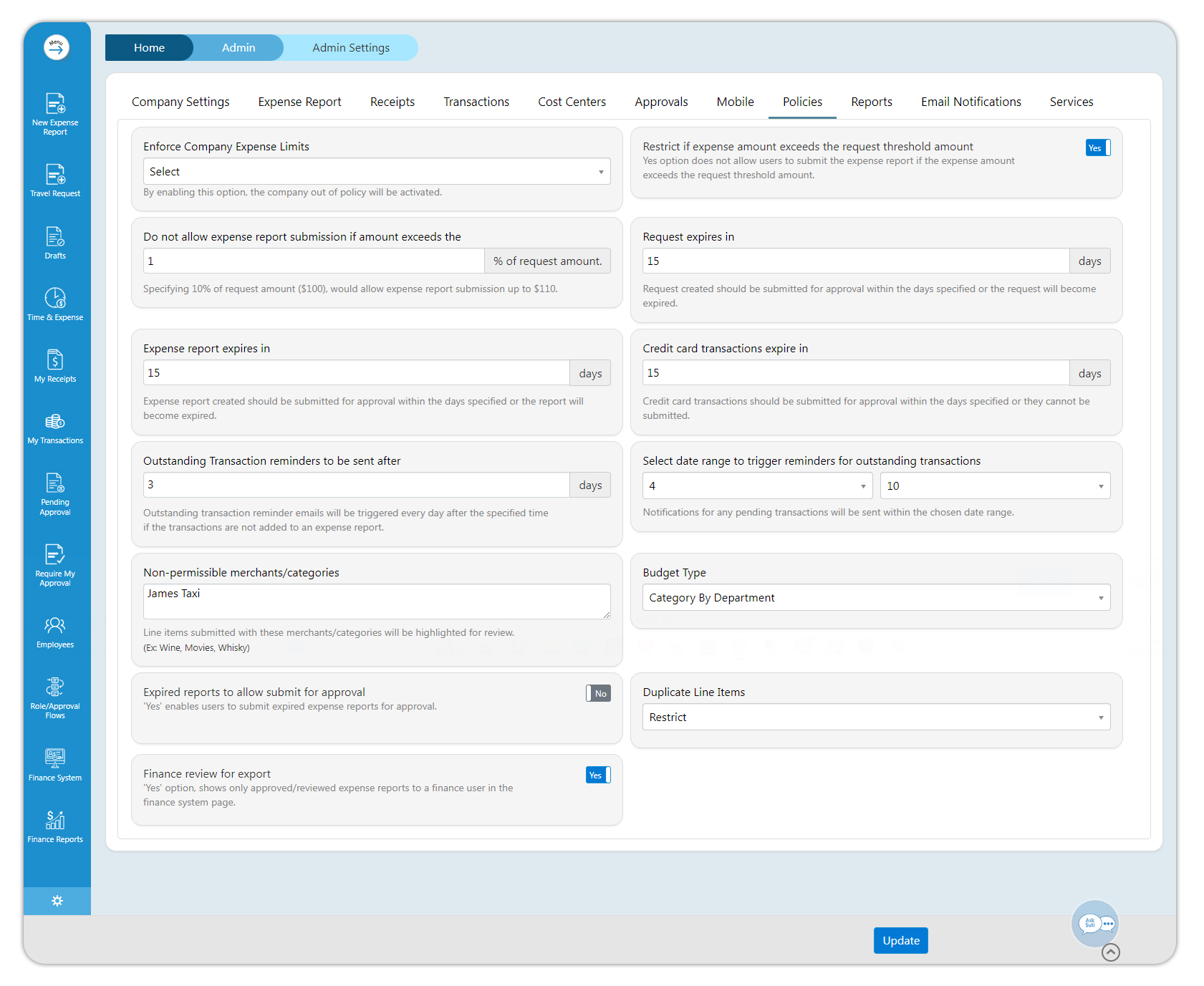This is a detailed screenshot of an admin page for an application or service, designed to manage expenses and budgeting for a business. On the left side, there is a vertical list of various categories set against a dark blue background. The categories listed include "New Expense Report" at the top, followed by "Drafts," "Time and Expense," "My Savings," "My Transactions," among many other options. The text in this menu is quite small, making it somewhat difficult to read.

The top of the page features a navigation breadcrumb with three links: "Home," "Admin," and "Admin Settings," indicating that the current page is "Admin Settings." The main content area has a white background with several tabs across the top for different subcategories, of which "Policies" is currently selected. 

Under the "Policies" tab, the page is filled with detailed information and settings related to expense policies. At the top left of this section, there is a heading that reads "Enforce company expense limits," accompanied by a drop-down box labeled "Select," which is currently not selected. Beneath this, there is a policy rule stating, "Do not allow expense report submission if amount exceeds," followed by a field indicating "percent of request amount," with a value entered as 1.

The remaining content on the page elaborates on various settings and regulations for handling expenses and budget constraints, providing administrators with the tools to enforce financial policies within the organization.